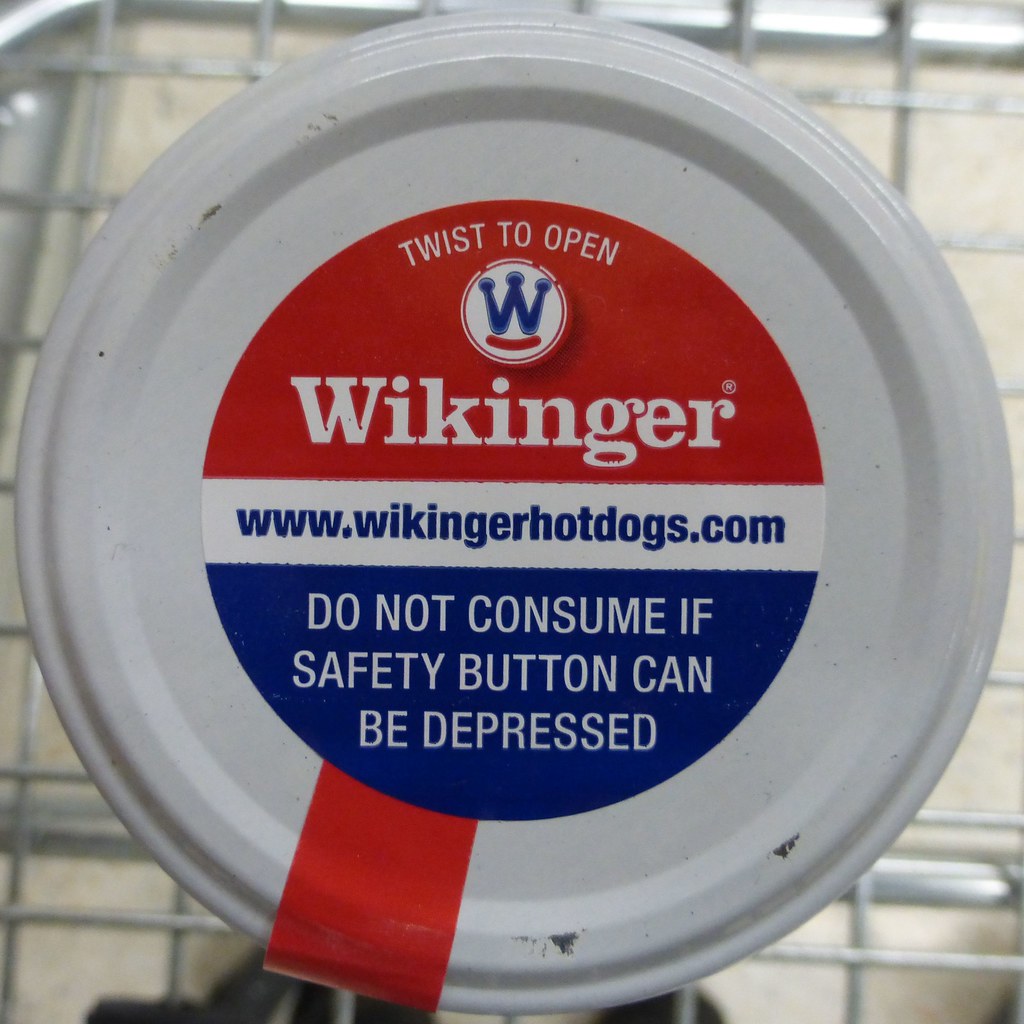The photograph captures the top view of a food package placed in a shopping cart. The package is a round, white container, distinguished by its label and safety seal. The container rests atop the metal grid of the cart, and the white tile floor of the store is visible beneath the cart. A round, two-toned label adorns the container's lid, with the upper half in red and the lower half in blue. Additionally, there is a prominent red sticker acting as a safety seal. This sticker, which ensures the container's integrity, carries the instructions "Twist to open" and includes a warning: "Do not consume if safety button can be depressed." The branding "Wikinger" is displayed on the label along with the website "www.wikingerhotdogs.com".